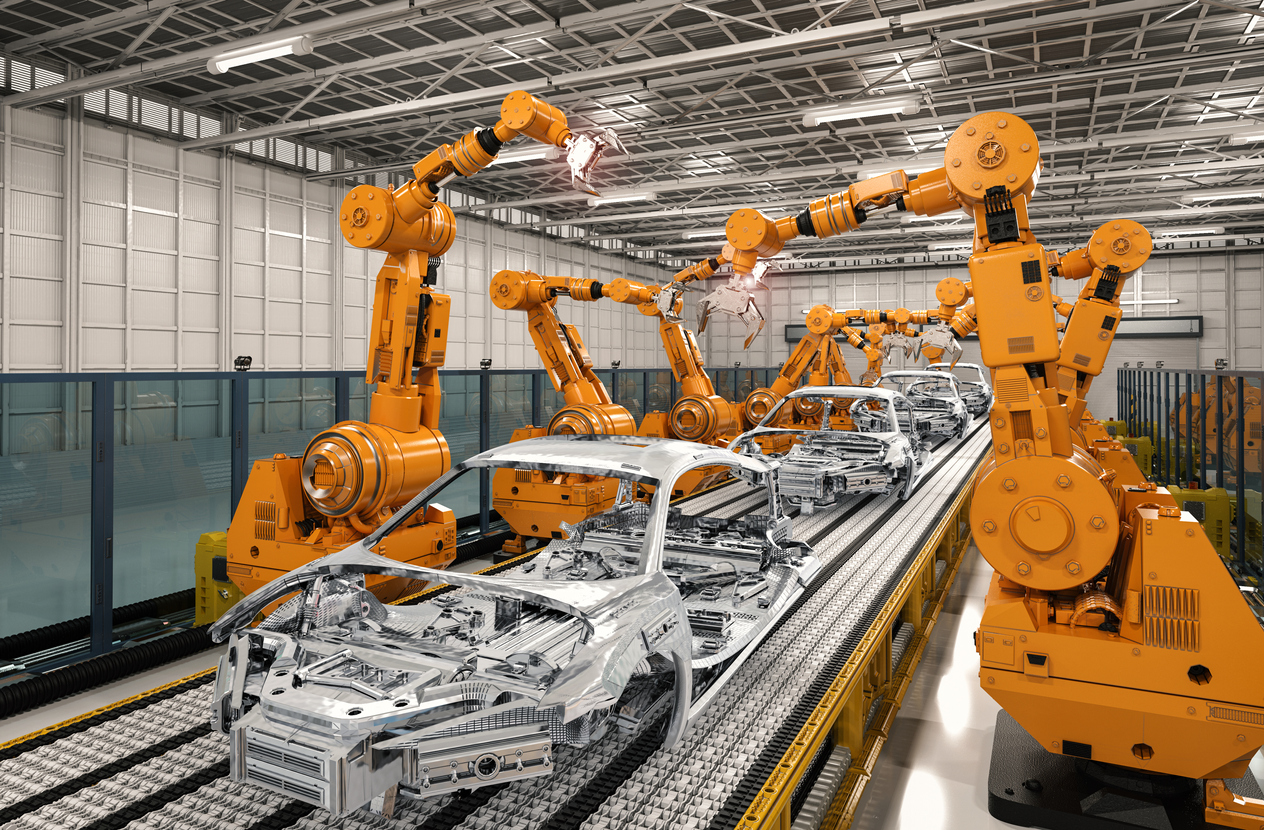The image captures an angled view of a bustling car factory, showcasing an assembly line where silver, half-constructed car frames are being meticulously crafted by a series of large, bright yellow and orange robotic machines equipped with mechanical claw-like arms. These robots are stationed in pairs along both sides of a wide, silver conveyor belt with bright yellow metal sides, extending across the industrial space. The building itself exudes a robust, utilitarian aesthetic with walls of half-white and teal colors accented by pervasive silver metal elements and beams, contributing to a stark, metallic ambiance. The ceiling is crisscrossed with silver trusses supporting long, rectangular fluorescent lights that illuminate the scene. Large green fences in the background add a contrasting color, while approximately a dozen robots, six on each side, execute different tasks to assemble the car frames.